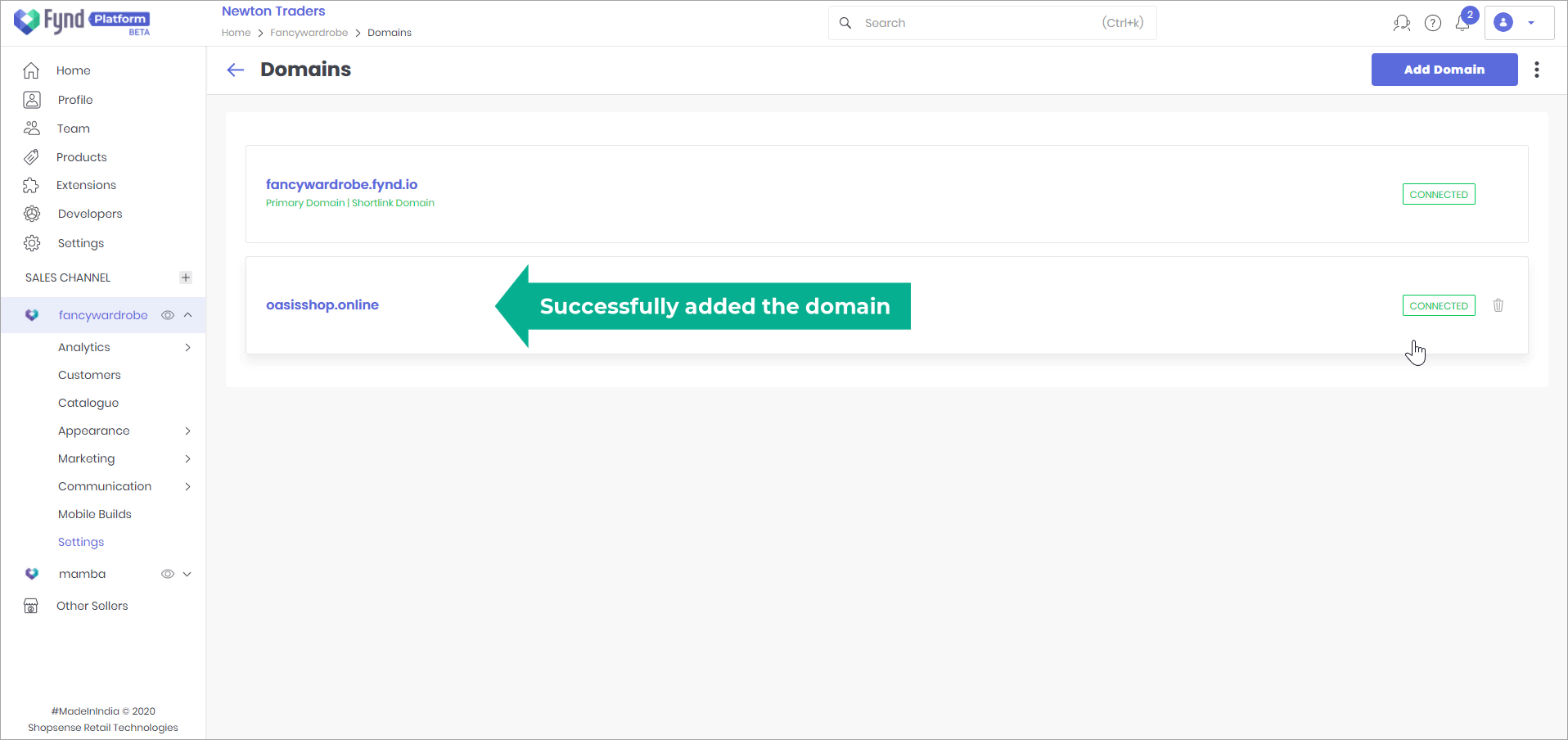A screenshot of a desktop displaying the FYND Platform application. On the left side of the screen, there is a vertically oriented menu featuring various options such as Home, Profile, Team, Products, Extensions, Developers, Settings, as well as a section labeled Sales Channel. Under Sales Channel, there are additional options including Analytics, Customers, Catalog, Appearance, Marketing, Communication, Mobile, and Settings.

The main panel of the screenshot is focused on the Domains section. Two domains are listed; the first is fancywardrobe.find.io, which is shown as connected. The second domain is oasisshop.online, which has a prominent green arrow beside it, indicating that the domain was "Successfully added." This area is identified as the "Add Domain" section, with a large blue "Add Domain" button located at the top right corner of the screen. The user interface appears clean and structured, guiding users through the process of managing their domains efficiently.